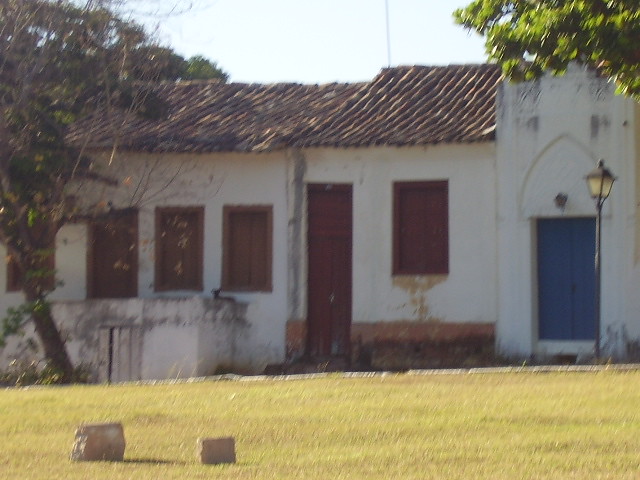The photograph depicts an older, possibly European building that seems to be well over 100 years old. The structure is primarily composed of white walls, resembling white concrete or stucco, and features a slightly pitched brown roof adorned with wooden shingles. The building is divided into two main sections with distinct entries: one section has a prominent blue door that resembles a tower with a vaulted arch, and a black streetlight nearby; the other section has a red door and several red-shuttered windows — three on the left of the red door and one to the right.

In the foreground, a large, flat grassy field stretches out, where a couple of large stones or statues lay, potentially indicating a cemetery in proximity to this historic structure. Vegetation is scattered around the edges of the building, with a tree visible on the right side and another partially hiding the left. The setting appears to be outdoors during the day, with a clear view of the sky above. The overall condition of the building appears quite run-down, suggesting that it might no longer be in use. The image is detailed in various colors including greens, browns, reds, blues, and whites, capturing a richly textured scene of this venerable edifice and its surroundings.